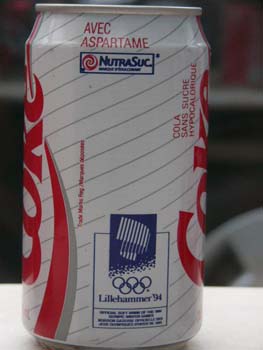This is a detailed, color photograph of a white Diet Coke can prominently featuring elements associated with the Olympics. The can is adorned with the iconic red Coca-Cola lettering and diagonal gray stripes. At the top, it reads "AVEC ASPARTAME" in red text, indicating the use of a sugar substitute. Below this, there's a blue rectangle that contains a NutraSweet logo, characterized by a white and red swirl design. Toward the bottom, the can has a reference to "Lillehammer 94," reflecting its association with the 1994 Winter Olympics. The phrase "coca-cola sans sucre hypocalorique" appears along the side, emphasizing its low-calorie nature. The can is placed on a white table, with a blurred, predominantly dark background enhancing the focus on the can.